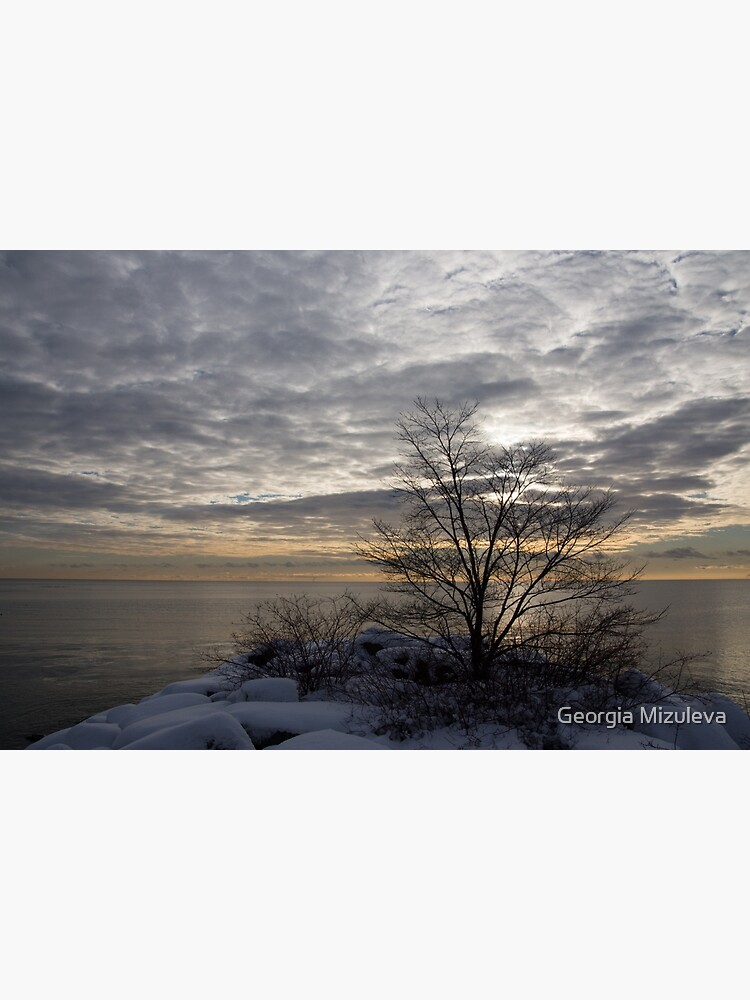Amidst a quiet, northern landscape at sunset, this remarkable photograph by Georgia Missouvia captures a snowy foreground where branches of out-of-season bushes and a small, leafless tree stand starkly against the soft, white terrain. This silhouetted tree and low brush add a haunting beauty to the scene. Beyond, a serene lake or ocean reflects the dimming light, while the sun peeks through a thick canopy of clouds, casting muted hues of yellow and blue across the horizon. The sky, dominated by dense clouds, lends a dark, somber tone to the entire image, highlighting the rugged, natural beauty of this tranquil setting. The photographer’s watermark, “Georgia Missouvia,” marks the bottom right-hand corner, adding a touch of personal signature to this evocative moment frozen in time.